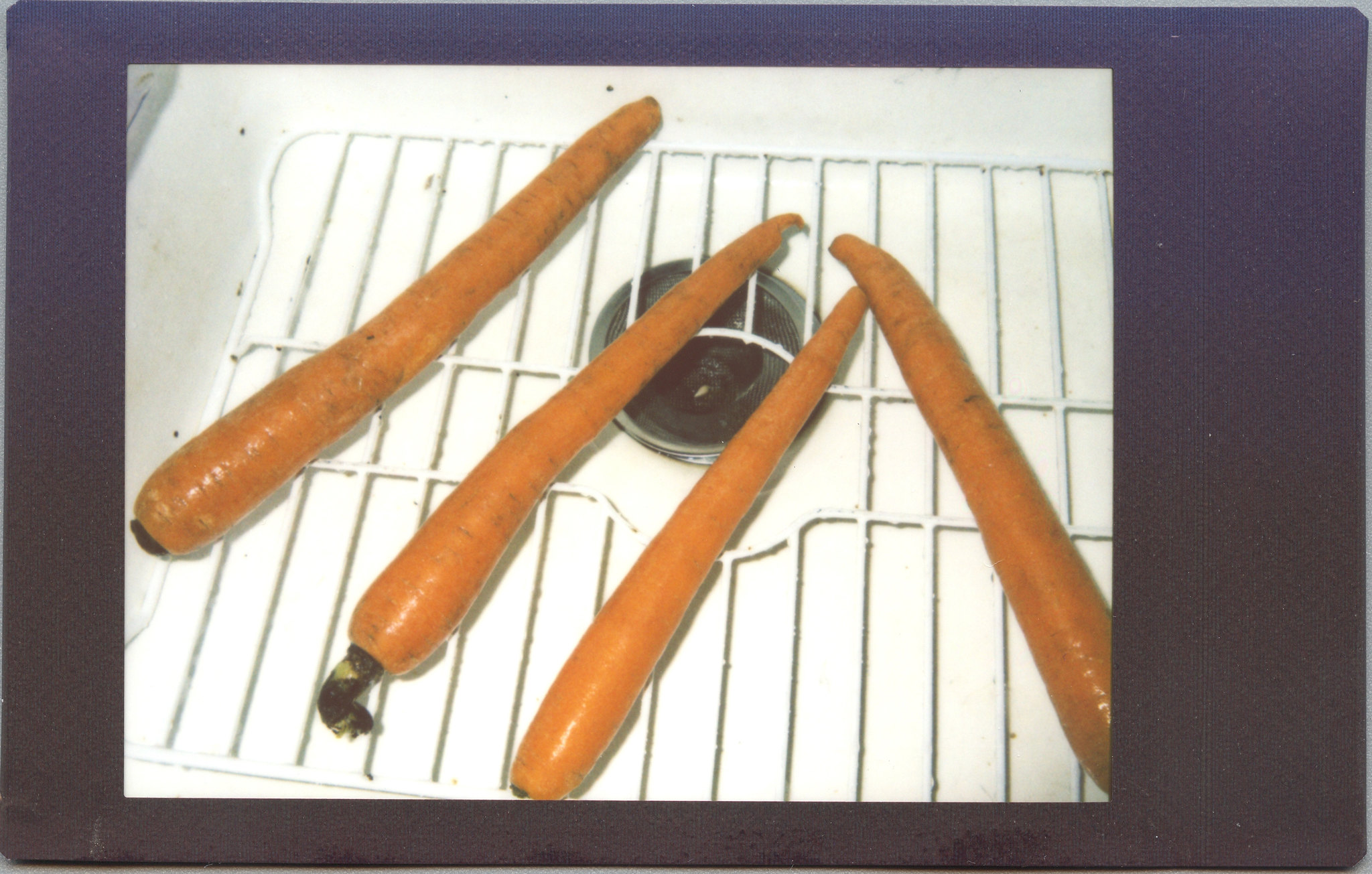This is a detailed photograph taken from above, showcasing four washed, unpeeled carrots lying in an old, slightly worn white kitchen sink. The sink includes a white wire drying rack with some vinyl peeling off, upon which the carrots are resting. In the middle of the sink is a circular drain with a black stopper. The carrots, all of a similar large size, have an orange glow and a wet appearance, suggesting they've been recently washed. The second carrot from the left retains a greenish-brown stem nub, while the others have had their stems entirely removed. The arrangement of the carrots is distinct: three lie diagonally from the bottom left toward the top right, and the fourth, positioned to the right, crosses over two of the others in a V-like formation. Some residual dirt on the carrots and small dirt patches in the sink hint that they still need to be scrubbed clean. The image captures this setup within a bordered purple frame, resembling a TV screen view.